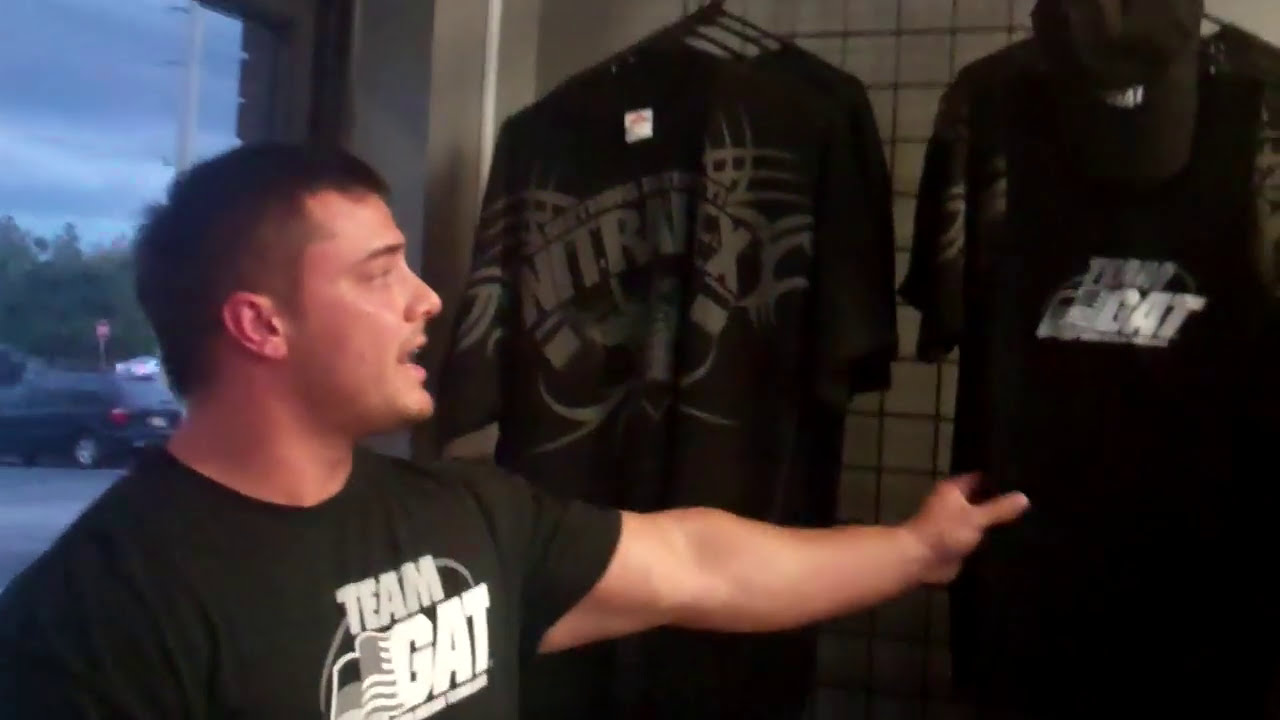The image depicts a Caucasian man with dark brown hair and slightly red-tinged skin, shopping in a store. He is wearing a muscular build and a short-sleeved black t-shirt that reads "Team G.A.T." in white letters, with "Team" in smaller gray letters above it. The man is reaching out with his left hand towards a similarly designed black t-shirt displayed on a rack, which also says "Team G.A.T.". The store has a light beige tile wall, and clothing racks holding multiple shirts, including one labeled "Nitrix," can be seen. In the background, a storefront window reveals a cloudy, rainy day with a few trees and a minivan parked in the lot. The man’s profile shows his open mouth, indicating he might be speaking.